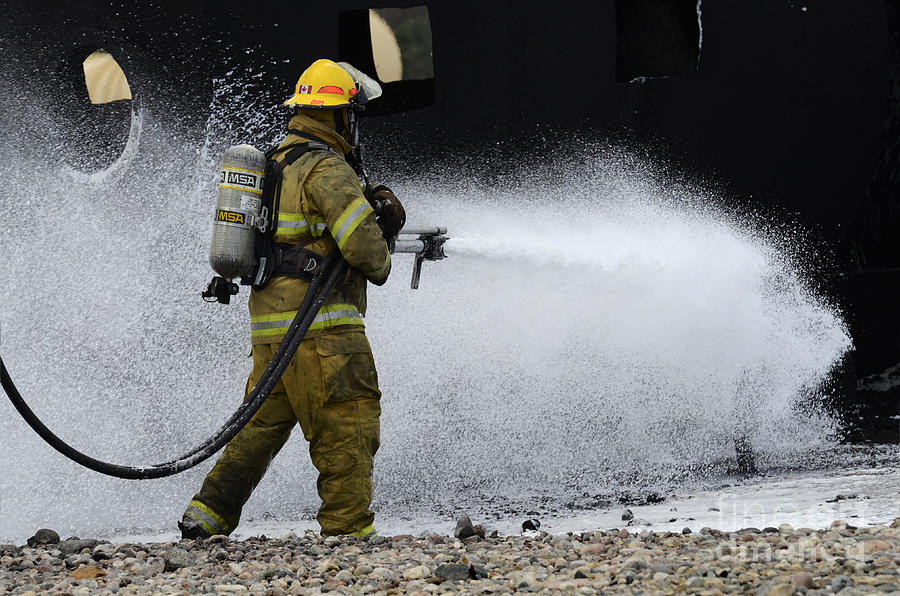A firefighter, dressed in a yellow protective suit and yellow helmet with an adaptable face mask, is operating a hose to spray water at what appears to be a burned area. The primary focus of the image is the heavy spray of water droplets, which obscures much of the background, making it difficult to discern the exact target. However, the dark, charred remains and square, rectangular shapes suggest it could be either a building or possibly an aircraft. The firefighter, slightly off-center in the frame, stands on a rocky ground that is drenched from the water, creating a large puddle around him. Strapped to his back are canisters labeled "MESA" or "MSA", likely indicating his breathing apparatus.